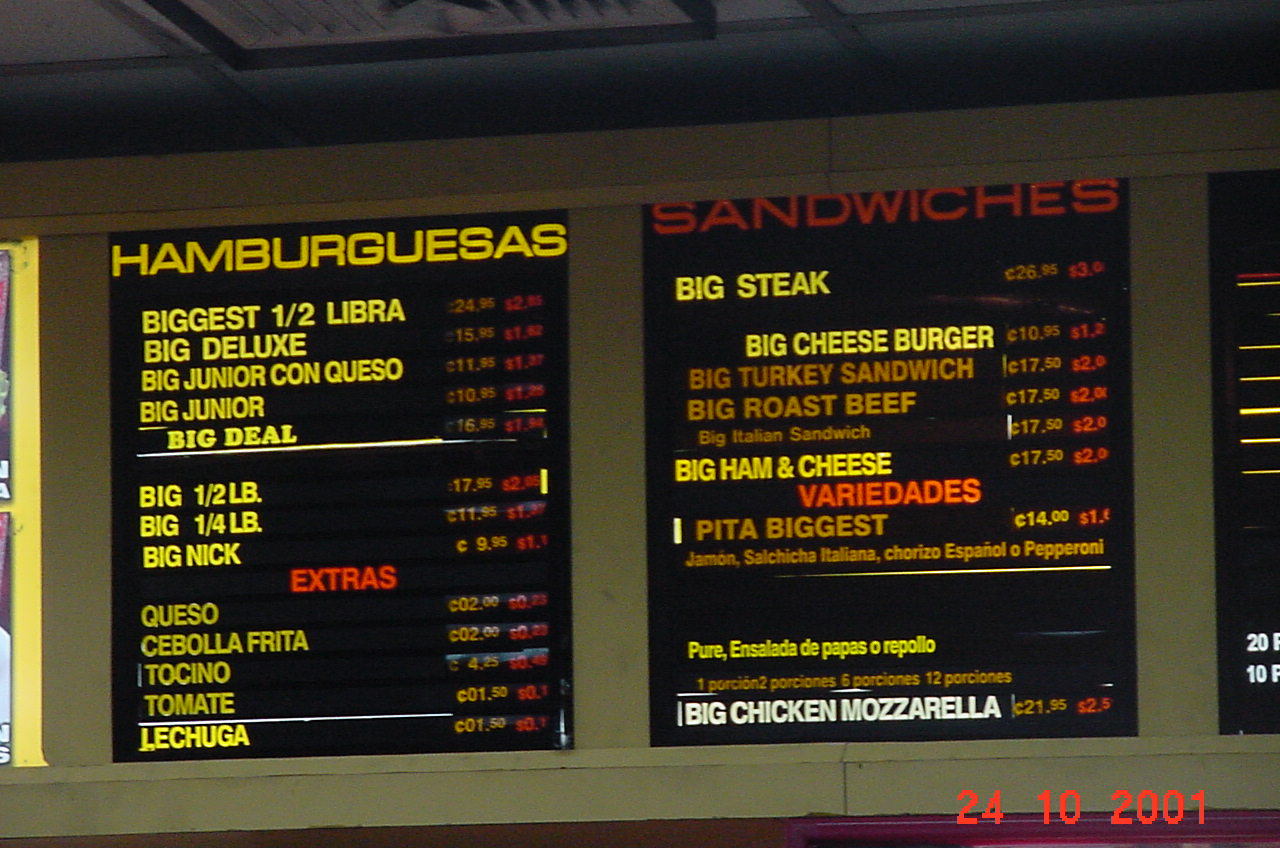The image depicts a menu from what appears to be a fast-food restaurant, dated October 24, 2001, in red numbers that read "24-10-2001" located at the bottom right corner. The menu features sections in both Spanish and English, indicating a bilingual offering. The background of the menu is predominantly black, providing a stark contrast for the descriptions and prices of the items. 

On the right side of the menu, under a red header labeled "Sandwiches," the listed items include:
- Big Steak
- Big Cheeseburger
- Big Turkey Sandwich
- Big Roast Beef
- Big Ham and Cheese Pita
- Big Chicken Mozzarella

The prices for these items are displayed adjacent to each description.

On the left side, which is in Spanish, the header is slightly unclear but seems to detail various burgers:
- Hamburguesas Biggs (Half Libra)
- Big Deluxe
- Big Junior con Queso
- Queso, Cebolla Frita, Tocino, Tomate, Lechuga

Each burger also has prices listed next to the descriptions. The image captures part of the tiled ceiling above the menu and a large gray border that separates the menu sections.